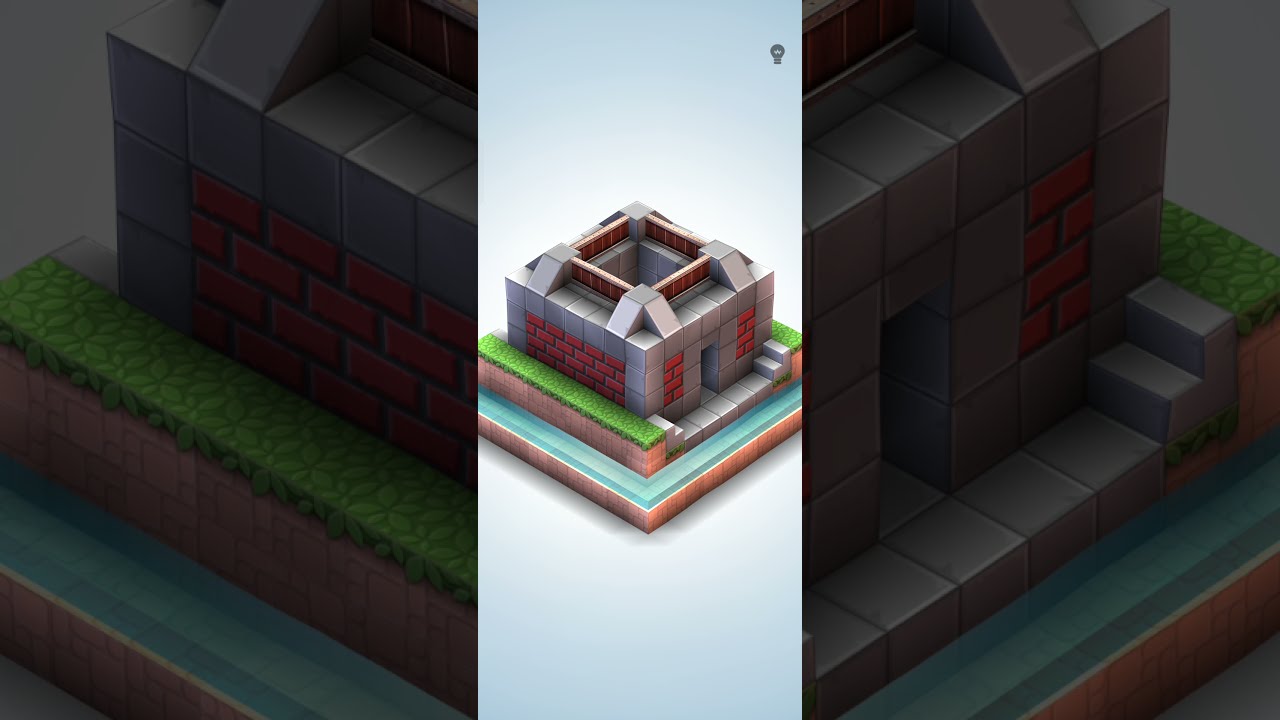The image is a computer-generated drawing of a blocky building reminiscent of Minecraft, displayed in portrait mode. The central building is constructed from red brick with gray stone pillars at the corners and features a square hole in its slightly raised roof, surrounded by a barrier, forming a mini balcony. The structure is bordered by greenery, including lines of grassy blocks with brown soil underneath, and incorporates concrete steps and gray blocks in front. Additionally, there appears to be a water channel encircling the building. The main image sits against a clear, whitish-gray background, with a small icon of a gray light bulb in the top right corner. This central image is framed by a zoomed-in, grayed-out version of the same building on the left and right sides, which enhances the focus on the main detailed building.